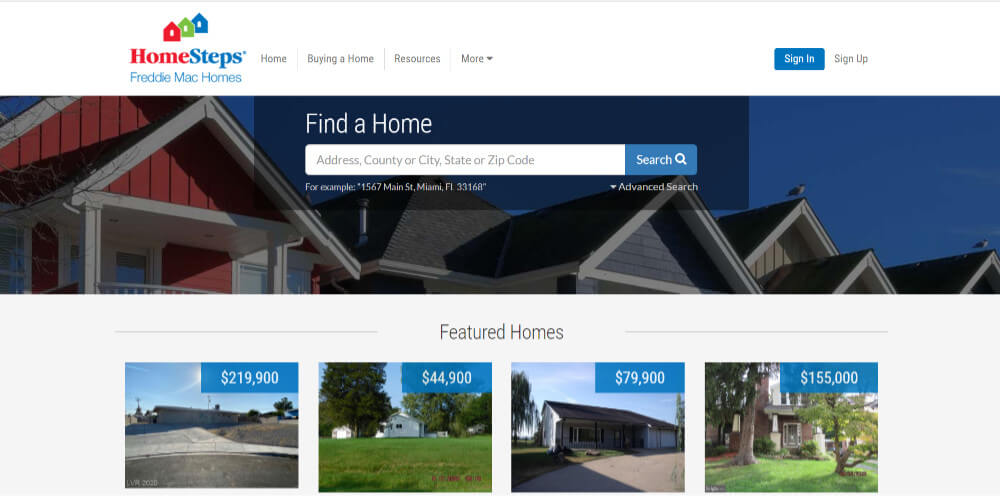The web page for Homesteps features a clean design with a prominent logo situated in the upper left corner against a white background. The logo depicts three overlapping houses arranged diagonally from right to left, colored blue, green, and red. Below the graphic, the text "Homesteps" is displayed with "Home" in red and "Steps" in blue, followed by the tagline "Freddie Mac Homes" in blue text.

To the right of the logo, a navigation menu offers four options in gray text: "Home," "Buying a Home," "Resources," and a "More" dropdown indicated by a down arrow. On the far right, a blue button with white text invites users to "Sign In," while a gray "Sign Up" option sits adjacent to it.

Beneath the navigation bar, a banner showcases a row of homes under a blue sky. The homes are uniformly shaped and colored red, blue, and tan. Notably, seagulls are perched on the roofs of the last two homes. 

Centered below the banner, the heading "Featured Homes" appears in gray text, flanked by decorative lines. Under this heading, four property listings are displayed as thumbnails, each with a blue price box in the upper right corner. 

- The first listing features a home viewed from the street on a sunny day, priced at $219,900.
- The second listing shows a small white home on a large green grassy lot surrounded by tall trees, priced at $44,900.
- The third listing presents a single-family home with a blue sky and some gray clouds above. It has a concrete round driveway and a moss-covered tree on the left, priced at $79,900.
- The fourth listing displays a home with a green front lawn, some trees, and a porch, priced at $155,000.